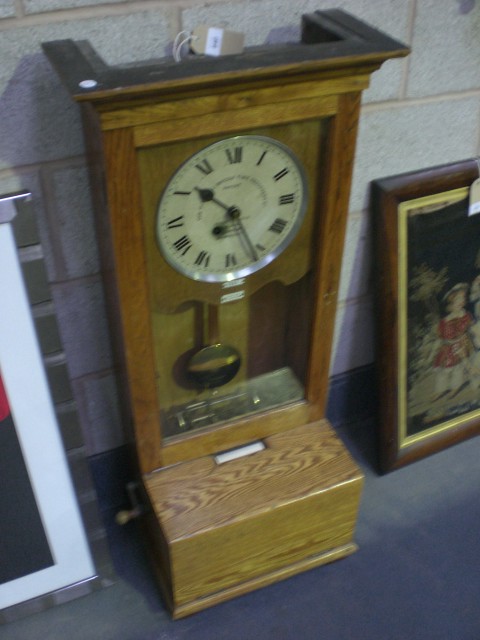In the image, we see a small, antique-style grandfather clock crafted from brown wood, set against a light-colored brick wall. The clock, which may be placed on a table or mounted on a wall, features a face adorned with Roman numerals and is complemented by hour, minute, and second hands. Surrounding the clock face is a wooden area approximately 10 inches long, extending into a decorative wooden box-like structure at the bottom, from which a gold circle hangs centrally. An adjustable handle is visible on the side of this structure, adding to its vintage charm. At the top of the clock, a brown price tag dangles from a string. Framing the clock, there are two photographs in frames—one positioned to the left and the other to the right. These items rest on a dark blue surface, enhancing the ensemble's visual appeal.